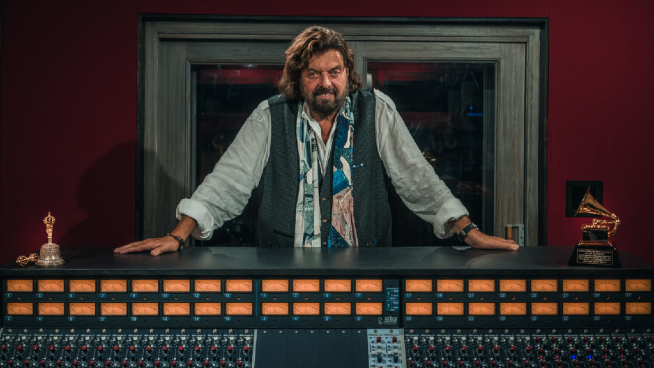This image depicts Alan Parsons standing in a dimly lit control room, prominently featuring a massive sound mixer with an array of knobs, lights, and buttons. Alan, an older musician around 50 years old, sports a long hair, a beard, a black vest, a loose white shirt, and a scarf. He has a watch on his left wrist and a bracelet on his right. Against a backdrop of a reddish wall, a large window frame or a big frame can be seen, along with a beautiful bell to his right and a phonograph, or gramophone, to his left. There are no visible texts, and the scene is bathed in colors of black, blue, gold, white, red, and gray. He stands upright with both hands on the sound mixer, appearing somewhat tired but relatively happy, presumably showcasing his awards amidst his sophisticated and atmospheric workspace.